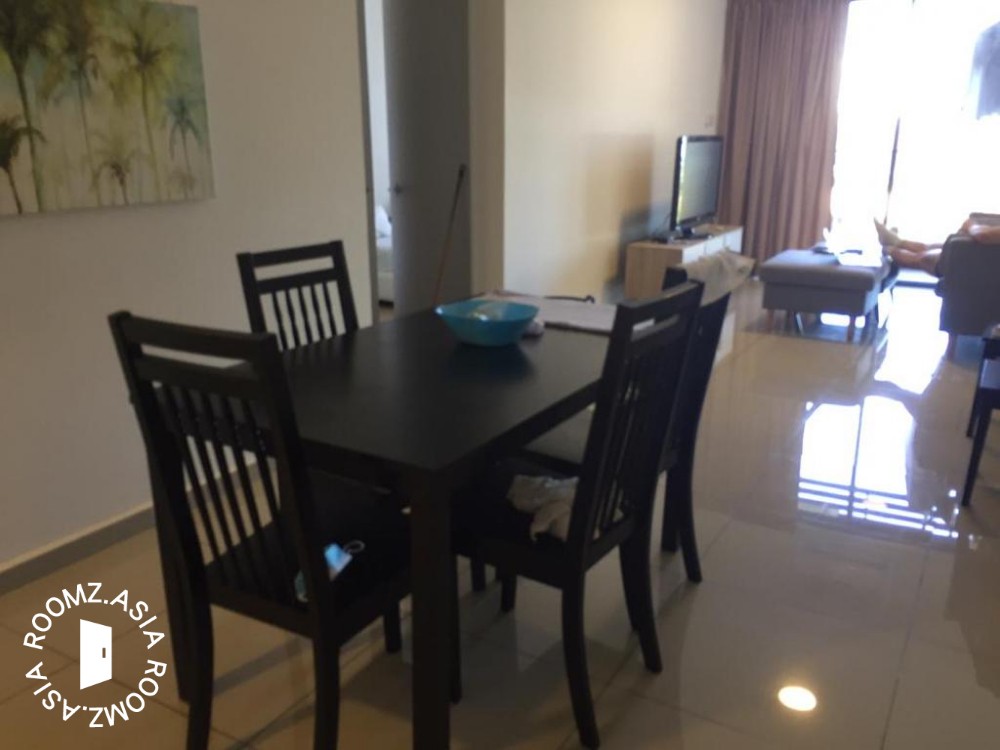A low-quality webcam photograph captures the interior of an apartment, branded with a "rooms.asia" watermark twice in the lower left corner, each with circular text and a door icon in the center. The floor is exceptionally shiny, reflecting a strong glare from sunlight streaming through the windows, which creates a strikingly bright highlight across the room. Centered in the lower portion of the image stands a black table paired with chairs; a blue bowl adorns the tabletop. In the background, a painting depicting trees and a natural scene embellishes the wall. Behind the table, a door is slightly ajar, adding depth to the composition. On the right side of the image, someone is seated, their feet propped up on an ottoman, facing a TV screen placed on a dresser. A long, pulled-aside purple or pink curtain partially reveals the window behind it, adding a touch of color to the scene. Notably, the pristine, glossy floor and the intense sunlight glare dominate the visual characteristics, further accentuated by a ceiling light's reflection in the lower right corner.